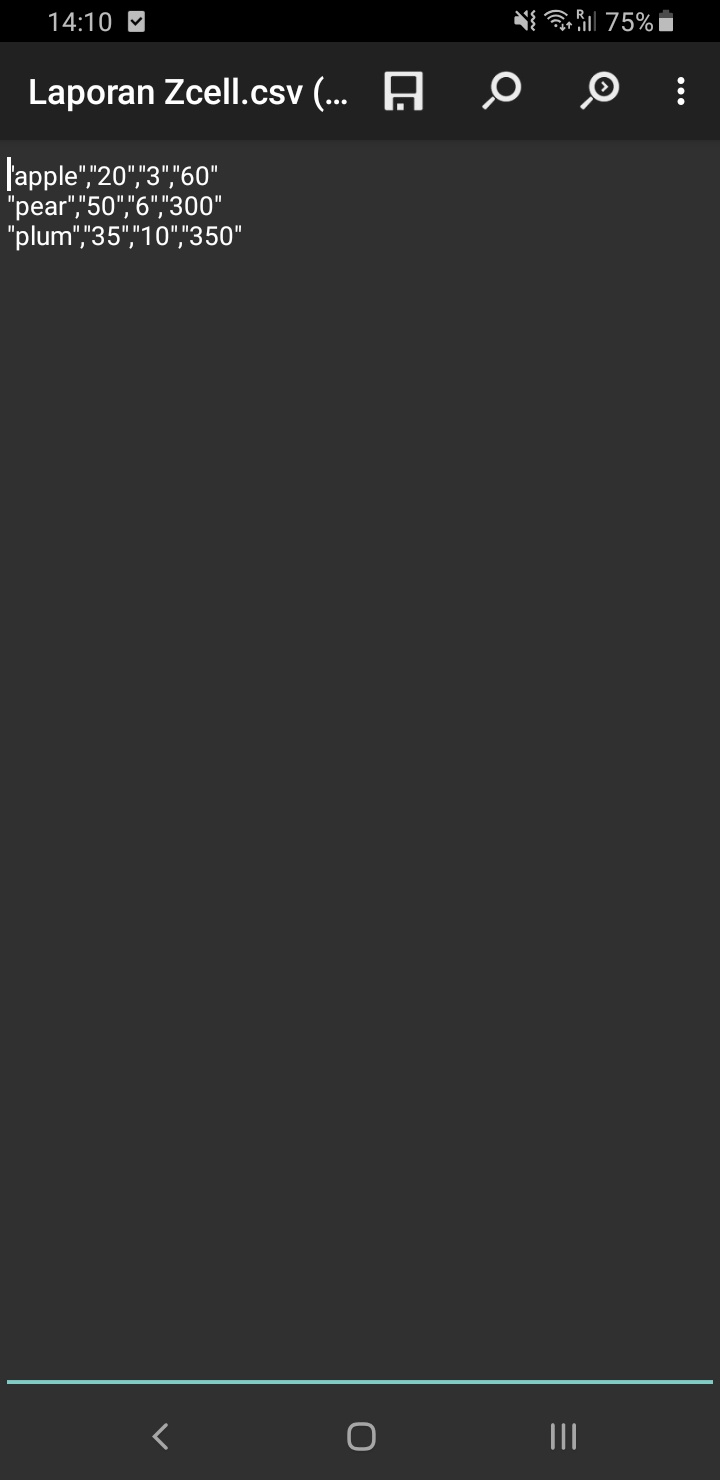The digital interface displays the time as 14:10 with a checkmark icon indicating a completed action. The WiFi signal icon shows three out of four bars and the battery level is at 75%. A file with the extension .CSV is referenced, accompanied by ellipses. A save icon is visible alongside a magnifying glass located on the right-hand side of the display. The word "Apple" appears in quotation marks, followed by the sequence "20", "3", and "60" also in quotations. Additionally, numerical values are listed: 50, 60, 300, 600, 35, 10, and 50.